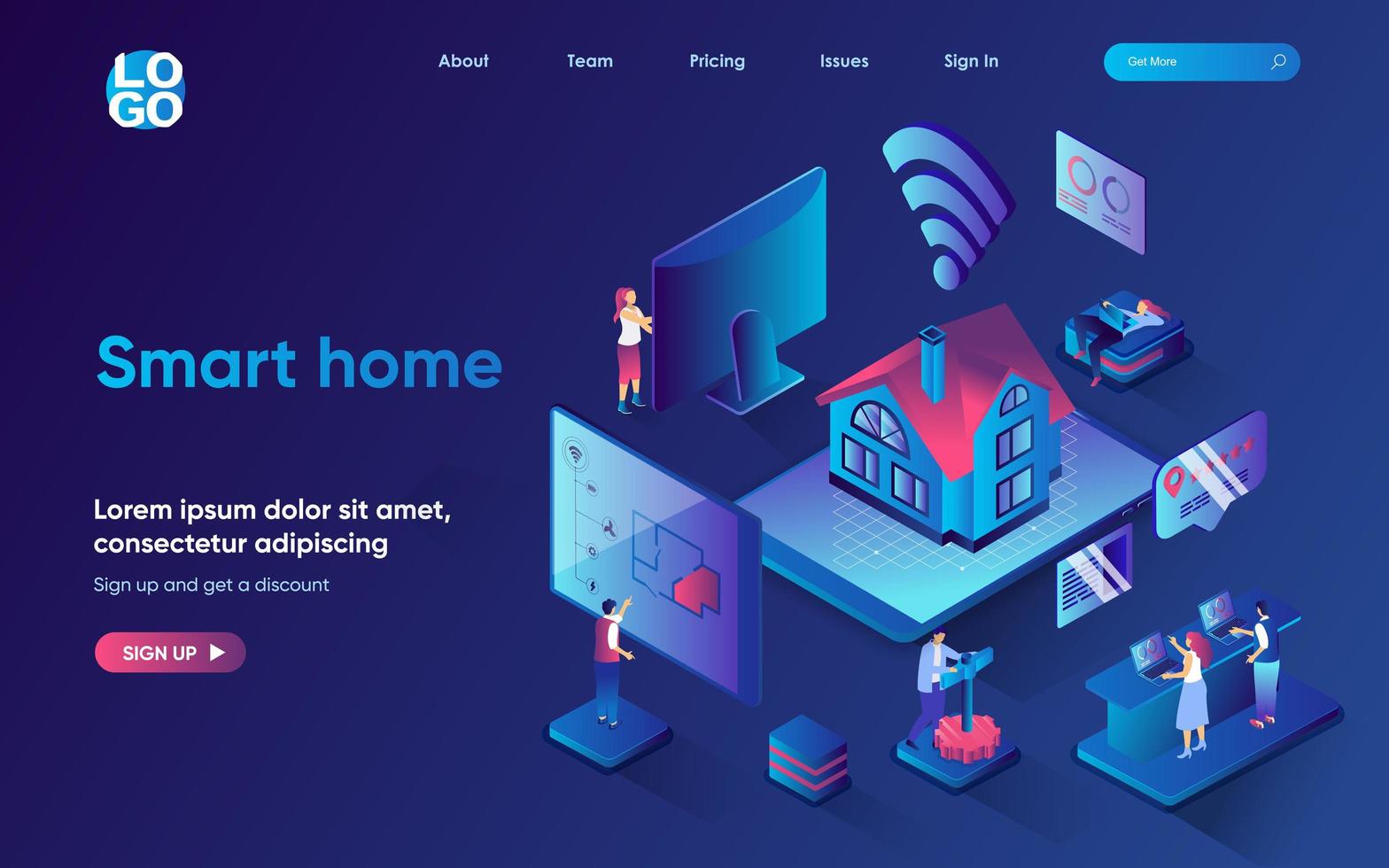This image depicts a vibrant website homepage for a smart home product. The background is a rich blue, capturing a blend between royal and navy blue. Prominently displayed in the top-left corner is a circular logo with the letters "G.O." in capital, accompanied by a stacked yellow design. Across the top navigation bar, options are listed: "About," "Team," "Pricing," "Issues," "Sign In," and a search bar labeled "Get More."

The left side of the screen features a bold "Smart Home" heading, followed by the text "Sign Up and Get a Discount" with a sign-up button highlighted in purple. Beneath this, smaller text includes additional sign-up instructions, partially in a foreign language.

Central to the image is a stylized, three-dimensional house on a platform, emitting a Wi-Fi signal from its chimney. Encircling the house, cartoon-like minimalist figures engage in various activities on laptops, computers, and phones. These figures illustrate different smart home functionalities, such as working on diagrams, lounging comfortably, and interacting with digital interfaces. Each character's action is visually linked to the house, emphasizing its role as the hub of a connected home ecosystem.